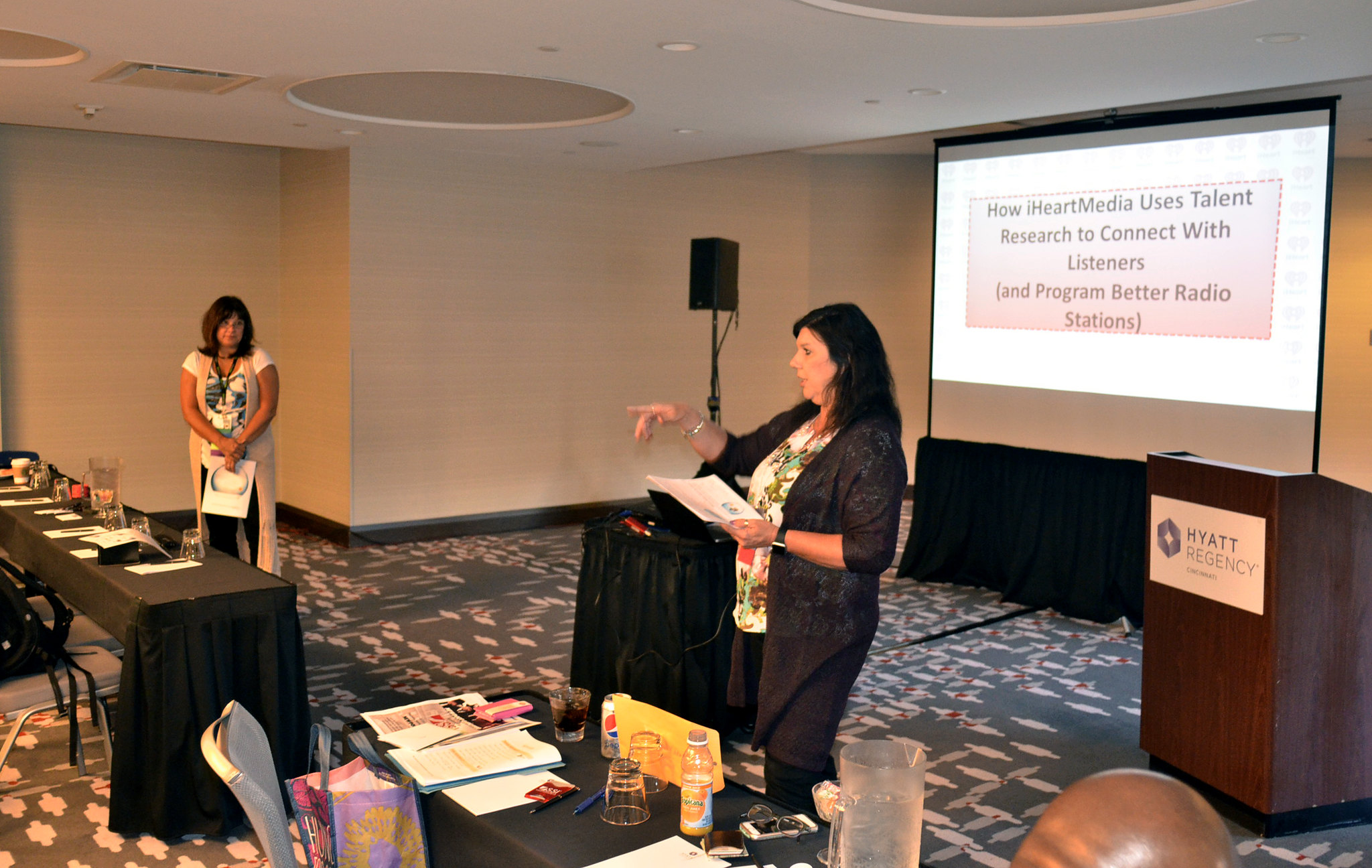The photograph is set in a bright conference room of the Hyatt Regency Cincinnati, featuring beige walls and lighter ceilings. In the center of the image stands a woman with long dark hair, wearing a multicolored blouse under a long coverall and dark pants. She holds a piece of paper in her left hand, gesturing to an unseen audience member while presenting. The PowerPoint screen behind her displays a slide titled "How iHeartMedia Uses Talent Research to Connect with Listeners and Program Better Radio Stations." Just a few feet behind her is a lectern. To her right (the viewer's left), another woman with long dark hair stands, holding a pamphlet and observing the speaker. In front of this second woman, there is a long black table cluttered with papers and containers. A similar table is positioned before the speaker, adorned with papers, glasses, bottles, and a water pitcher. The audience space appears mostly empty aside from a visible hand in the far corner and the back of a bald head in the lower right, underscoring the sparse attendance.